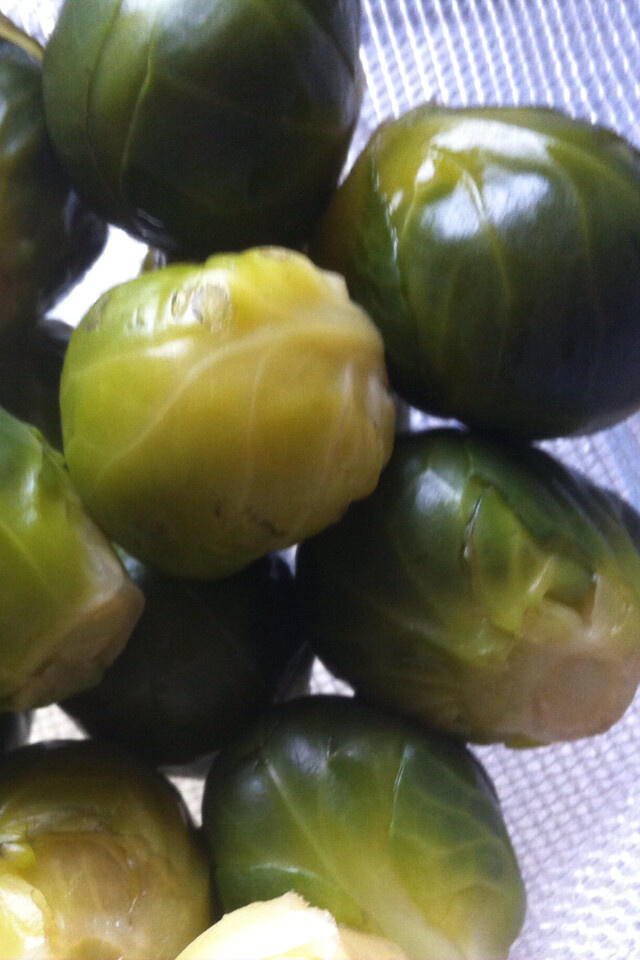This is a very close-up photograph of approximately 10 or 11 Brussels sprouts, tightly clumped together and resting on a bright white surface that appears to be either a paper towel or a woven, mesh-like dishcloth. The white background features a textured pattern with crisscrossed lines. The Brussels sprouts exhibit a mix of colors, from dark green to light lime green, and demonstrate a noticeable shininess, as if illuminated by overhead light. Some sprouts reveal their cut stalks, while others show a bit of yellowing alongside their varied green hues. The arrangement is somewhat jumbled, with the sprouts closely packed, allowing glimpses of the white background to show through in the spaces between them. The clean and healthy appearance of the Brussels sprouts makes them look ready for use, possibly as a garnish or in a salad.